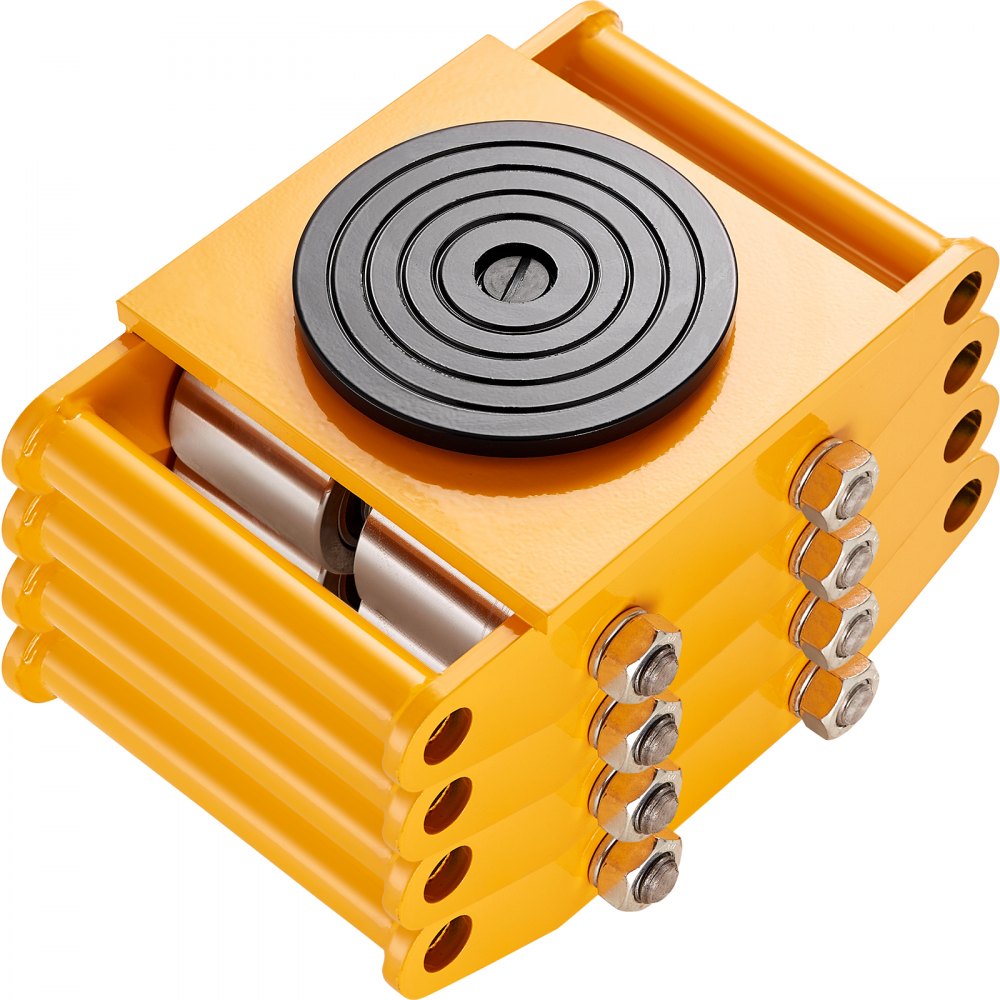This color photograph features a square-framed image centered on a piece of metal equipment, likely a jack or lift, viewed from above. The equipment consists of four distinct levels made of bright yellow metal with large silver bolts. The structure is designed to extend like an accordion, with several metal parts visible in the middle. The top of the equipment is a black, circular, textured surface that resembles a turntable. The body is composed of yellow metal segments with silver metal components inside and additional metal screws. The overall style of the image is a product photograph, highlighting the intricate details and colors—yellow, silver, black—of the tool.